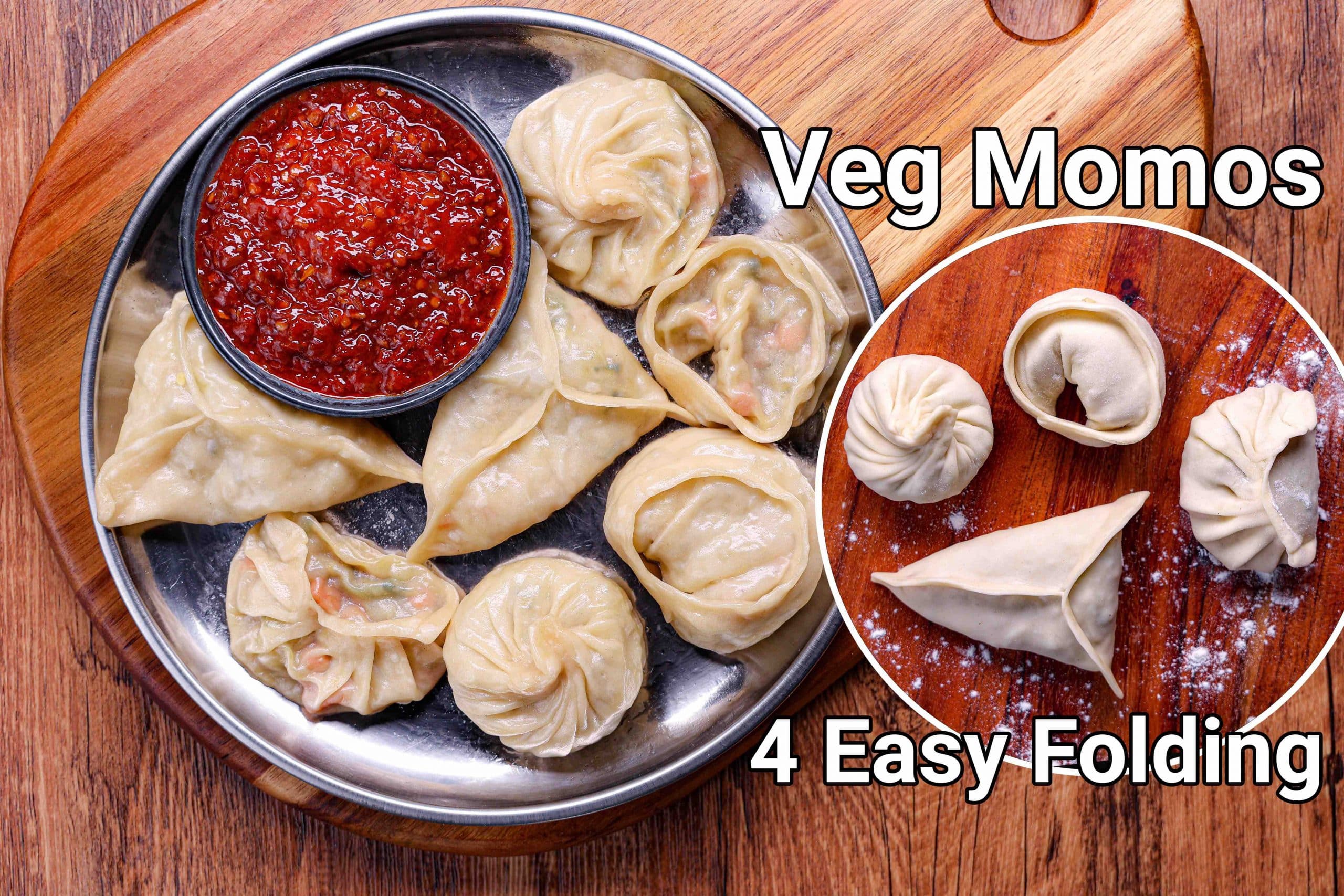This photograph, taken from a top-down view, captures a wooden table featuring a striking array of food items on display. Centered on the left side is a large, silver-colored, metallic plate which holds a black-rimmed bowl filled with a chunky, red dip sauce. Surrounding the bowl are several pieces of moist-looking momos, yellowish in hue and wrapped with visible vegetables inside. On the right, there is a white, circular element, likely a digitally added image showcasing more momos, these appearing noticeably drier. The circle has a background text in big white letters spelling out "VEG momos" and below it, a smaller caption stating "for easy folding." The entire setup rests on a brown wooden table characterized by streaks of light wood in hues of white, yellow, and orange, contributing to the warm tones of the image.